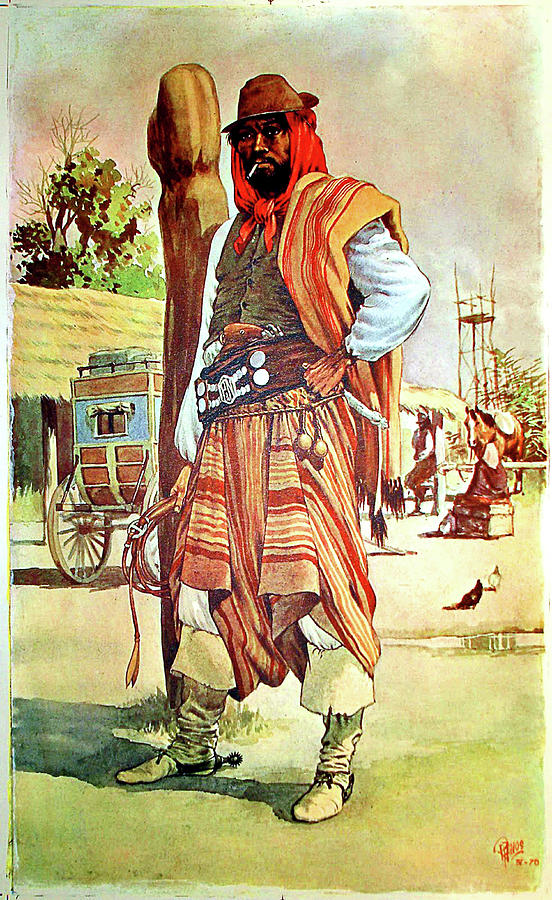This detailed drawing captures a black man from the Old West, richly adorned in era-specific attire. He wears a cowboy hat, accented by a red scarf wrapped underneath, and has a lit cigarette in his mouth. His facial features are rugged and weathered, indicative of someone familiar with frontier life. His attire includes a long-sleeved white shirt, a vest, and a flowing, blanket-like garment draped over his left shoulder, with red, blue, and white stripes. He has baggy pants tucked into white leather boots and a significant belt around his waist. His right hand firmly grips a whip, while his left hand rests on his hip, clutching a knife and a holstered gun. The background paints a vivid scene with a wooden post, likely for tying horses and buggies, a stationed carriage, several horses, and other figures casually leaning on fences. Birds are seen in flight and a solitary figure sits on boxes, rounding out this evocative portrayal of the period.